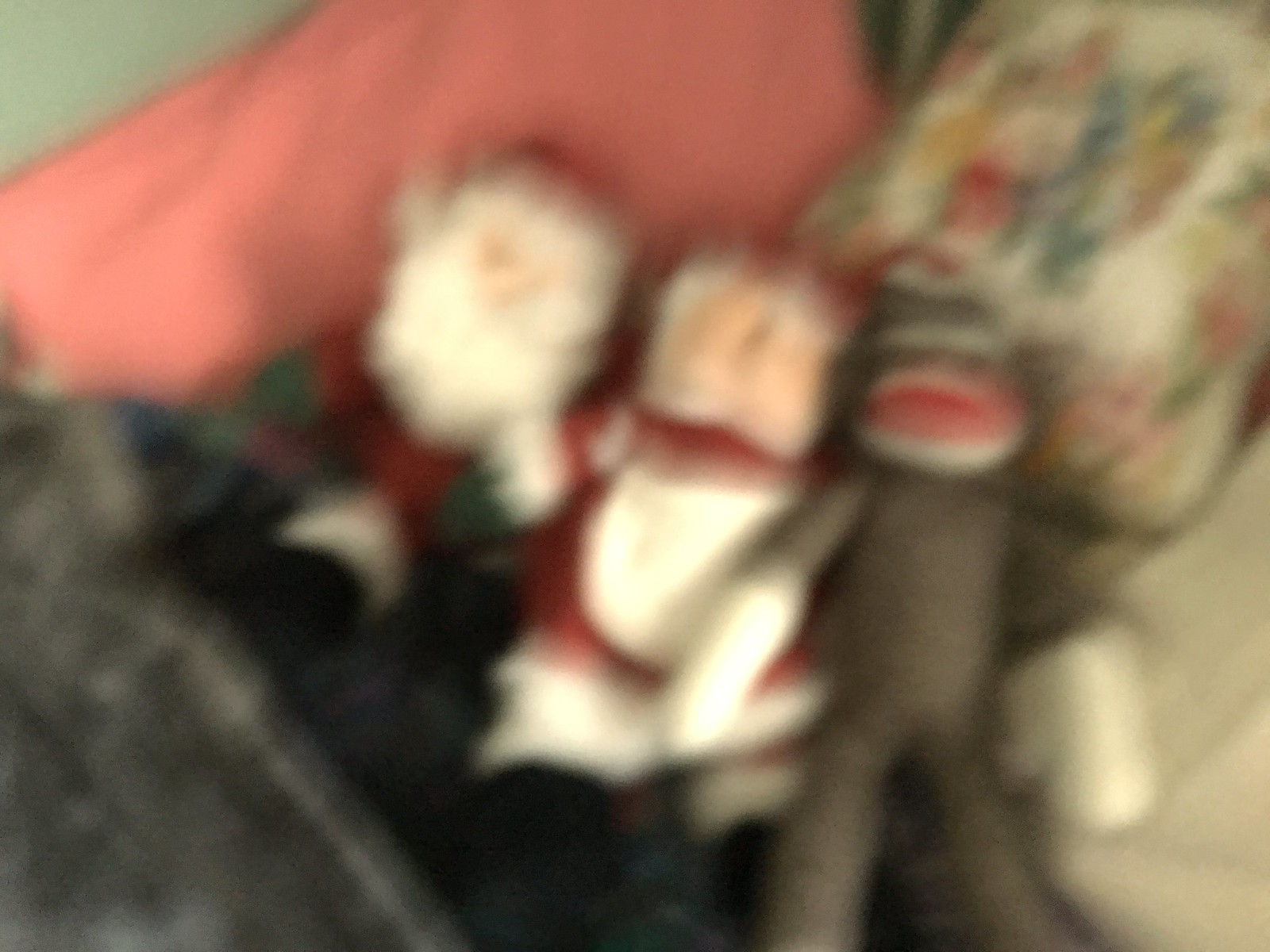This extremely blurry photograph appears to depict three stuffed dolls situated on a gray blanket with multiple throw pillows behind them. In the center of the image are Mr. and Mrs. Claus dolls, both dressed in red suits with white accents and black boots. Mrs. Claus, positioned in the middle, is wearing a white apron over her red dress, while Mr. Claus, to her left, sports a red hat along with his iconic white beard. On the right side is a sock monkey with a brown body, red mouth, white mitten-like front paws, and a knit cap. Above the monkey is a floral throw pillow, while a coral-colored square, possibly another pillow, is seen above the Clauses. The lower left-hand corner of the image shows a gray object, though its details are indistinguishable. The photograph seems to have been taken with a cell phone camera in motion, contributing to the overall blurriness.